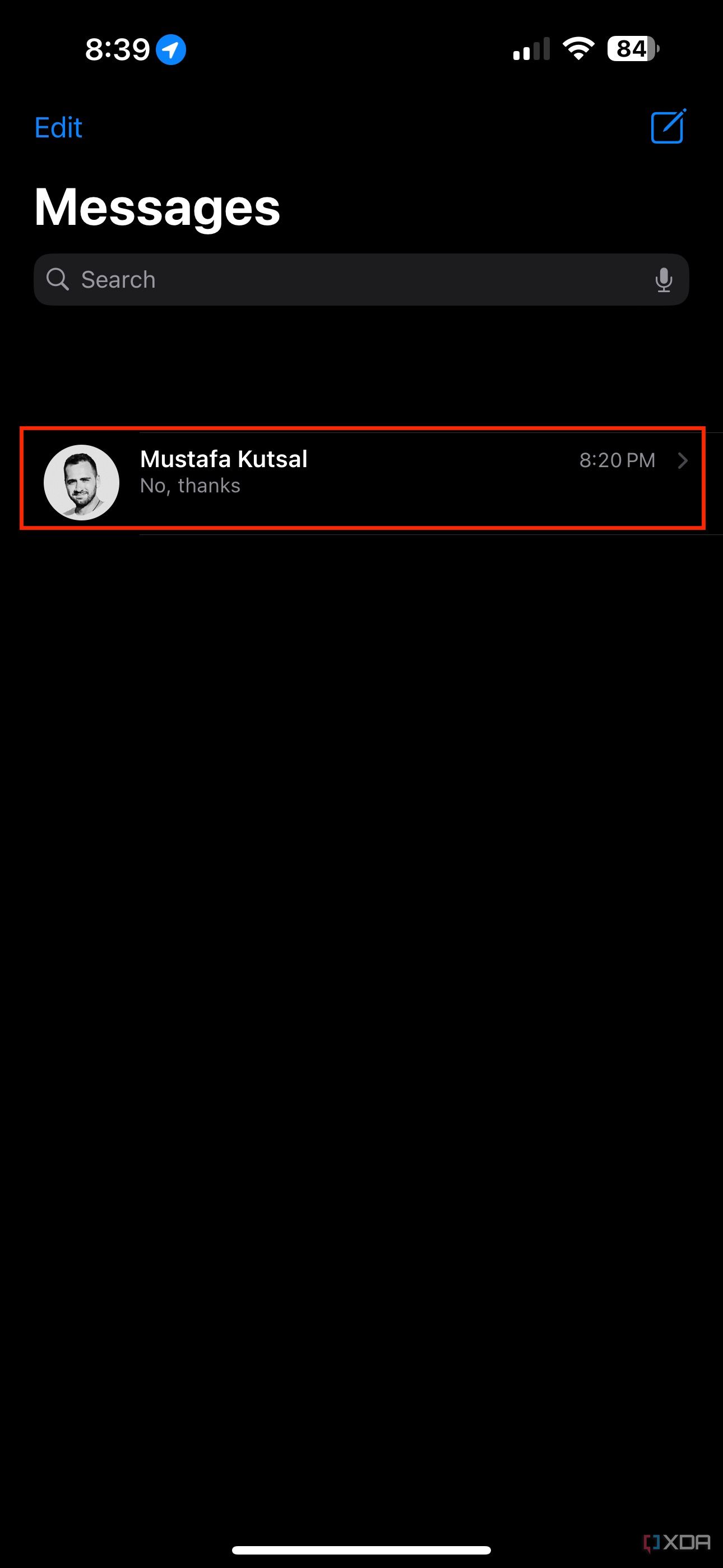In this image, there is a screenshot of a mobile device interface. At the top left corner, the time is displayed as "8:09." Directly to the right of the time, the WiFi signal strength icon is visible. On the opposite side, in the top right corner, the network signal bar is shown, indicating the device's connectivity, next to a battery level indicator showing 84% charge remaining.

The main portion of the screen features a text editing interface. The header reads "Edit Messages,” with the name "Mustafa Kutsal" prominently displayed in the middle, highlighted in red. Below, there is an option labeled "No thanks," contributing to the status of the messaging interface. Additionally, there is a timestamp stating "8:20 PM."

The overall color theme of the screen is black, providing a stark contrast to the text and icons. Finally, in the bottom right corner of the image, the text "XDA" can be seen in small print, marking the affiliation or source of the device or screenshot.